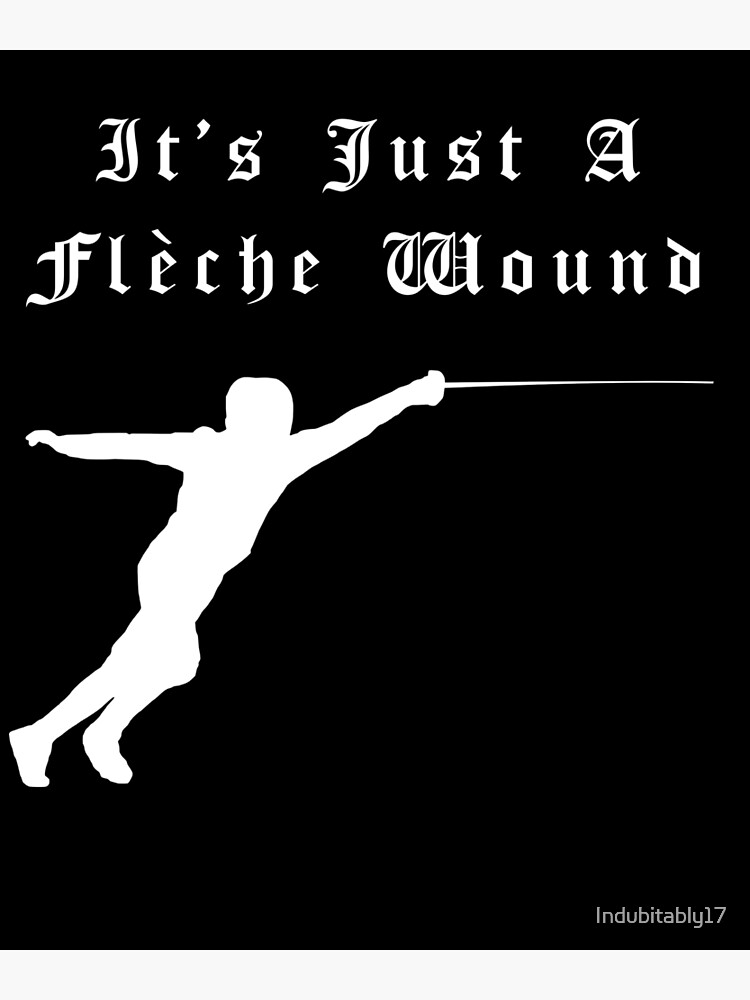The image is a minimalist digital art piece, roughly the size of a sheet of paper but slightly shorter. It features a striking white silhouette of a fencer lunging forward against a pure black background. The fencer's right arm is extended, holding a rapier that points horizontally. Near the top of the image, in an Old English-style font, are two lines of text that read: "It's just a flèche wound." Notably, "flèche" is spelled F-L-E-C-H-E, with a downward-sloping apostrophe over the first "E." Additionally, there is a discreet watermark in the lower right corner that reads "Indubitably 17."